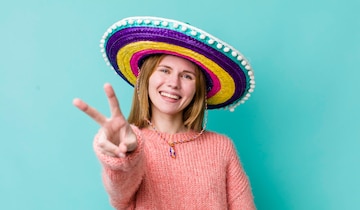The photograph depicts a young, smiling woman with a light complexion, framed by a solid turquoise blue background. She's facing the viewer and sporting a distinctive sombrero adorned with various stripes of color: the outermost ring is teal, followed by deep purple, then an orange or yellow, leading to a hot pink ring nearest her head. White tassel balls hang from the teal brim, adding a festive touch. Her blonde or possibly light red hair is styled in a shoulder-length bob. The woman is dressed in a long-sleeved, ribbed sweater of a salmon or pink hue. Her playful demeanor is captured by her one hand down and the other extended towards the camera, flashing a peace sign. The photograph ends around the middle of her chest, highlighting the top portion of her torso and the sombrero's strings draped around her neck like a necklace. Despite the small size of the image, the details of her smile, showcasing her white teeth, and possibly blue eyes are evident.